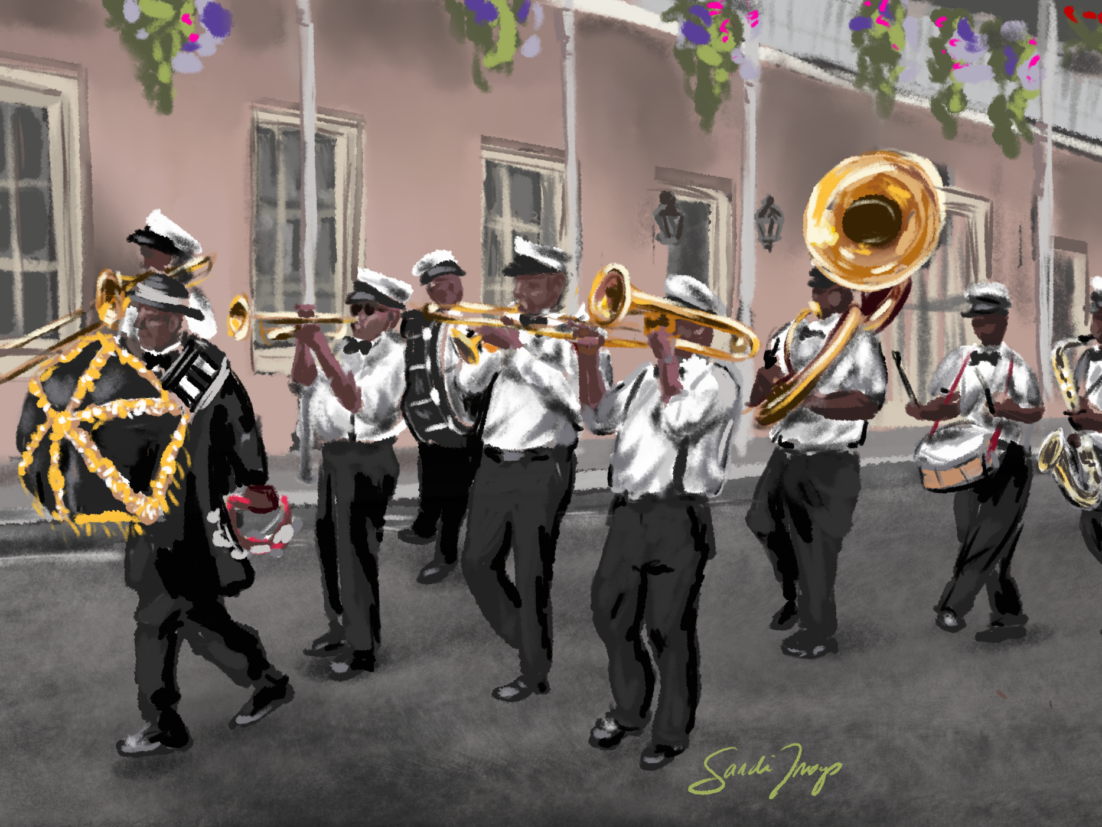This is a stylized and slightly blurred painting of a marching band parading down a city sidewalk in New Orleans. The band members are dressed in coordinated uniforms featuring black pants, white long-sleeved shirts, and a mix of bow ties and suspenders. The front figure, possibly the Grand Marshal, stands out in an all-black outfit complete with a hat and jacket, and he carries a tambourine in his left hand and a black umbrella adorned with gold trim. The parade includes musicians playing the trombone, trumpet, tuba, bass drum, snare drum, saxophone, and bugle. The background reveals a pink building with balconies decorated with colorful flowers, evoking a festive New Orleans atmosphere. The road they march on is gray, and at the bottom of the painting, the artist's signature reads "Sandy Tway."